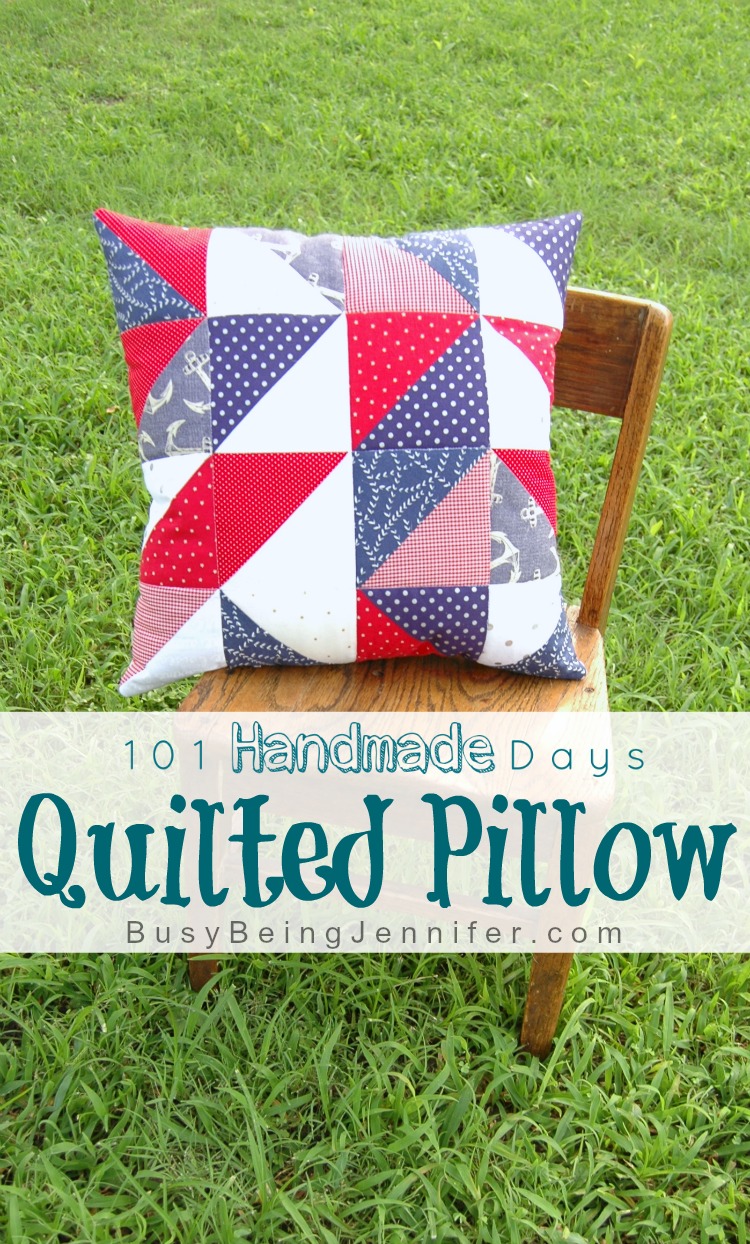A vibrant green lawn, in need of a trim, serves as the backdrop for a charming scene featuring a small wooden chair with a quilted pillow atop it. The pillow, a creation showcased on BusyBeingJennifer.com as part of the "101 Handmade Days" project, is a beautiful, intricately designed piece. It features triangles and half-square patterns predominantly in shades of red, white, and blue. Some tiles display polka dots, others solid colors, while some boast whimsical swirls and anchor motifs. This vibrant combination of patterns and colors gives the pillow a distinct, lively charm. A white sign draped across the chair showcases the text "101 Handmade Days Quilted Pillow" in Comic Sans-like blue letters, with "BusyBeingJennifer.com" noted below in smaller text. The overall composition highlights the rich texture and artistic craftsmanship of the quilted pillow against the earthy simplicity of the wooden chair and lush green grass.